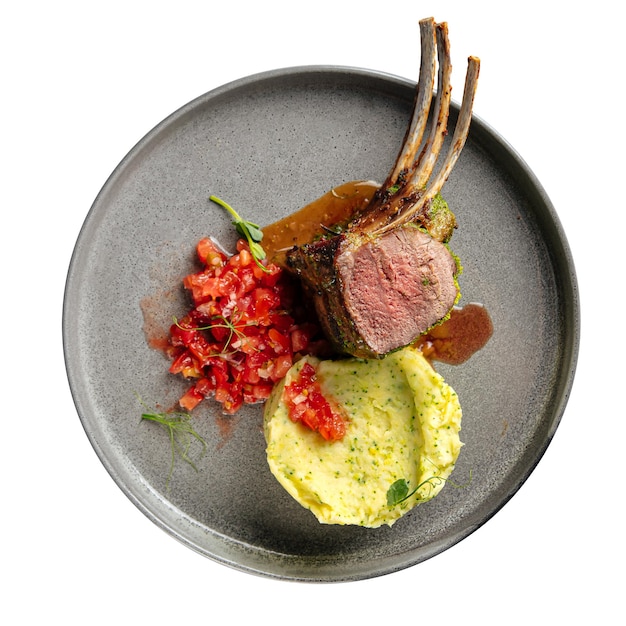The image is a color photograph taken from directly above, showcasing a meticulously plated dish on a ceramic plate with a gray and speckled appearance, featuring a high rim. The dish rests on a white background. The focal point of the dish is a trio of frenched lamb chops positioned in the top right quadrant, exhibiting a beautifully rare, pink interior and seared brown edges, bathed in a translucent brown sauce. Adjacent to the lamb chops, on the left side of the plate, is a salsa-like relish made of diced tomatoes, speckled with green herbs, possibly parsley, and hints of garlic. Below the lamb chops, in the lower right section of the plate, is a yellow pat of what seems to be a cooked egg or mashed vegetable, interspersed with green flecks. The overall presentation is embellished with sprigs of green, adding a fresh contrast to the rich, colorful components of the dish.